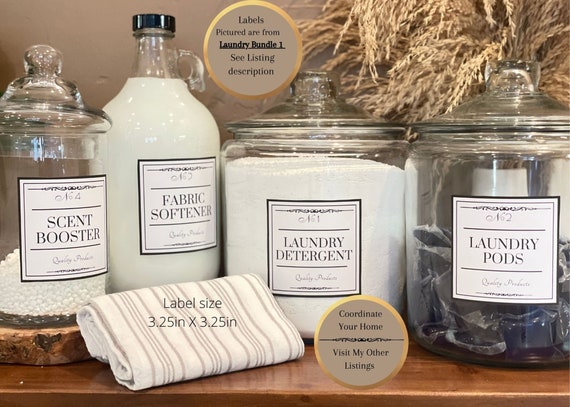This indoor photograph captures an elegant and organized laundry setup displayed on a table. It features four different glass jars and bottles, each with a clear, hand-printed label. The jar on the far left contains scent booster pods and is labeled "Scent Booster." Next to it is a large jug with a black cap filled with liquid fabric softener, bearing a label that reads "Fabric Softener." The third clear canister holds laundry detergent, while the final jar stores laundry pods. All labels are designed in a white and black color scheme for a cohesive look. In front of the assemblage, there is a folded white and gray striped hand towel adding to the aesthetic appeal. The photo also includes a circular label at the top that reads, "Labels pictured are from Laundry Bundle 1. See listing description," with a similar label at the bottom encouraging viewers to "Coordinate your home. Visit my other listings." This setup promotes an organized and visually pleasing way to store laundry essentials, ideal for those looking to add a touch of sophistication to their laundry room.